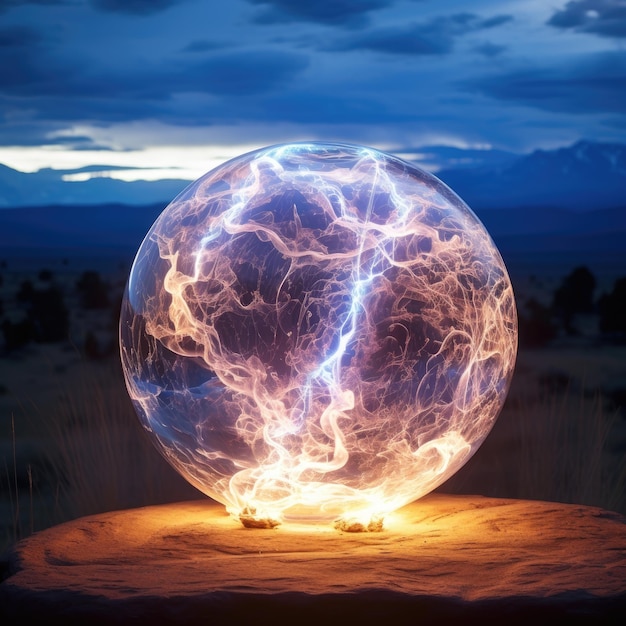In the image, a fantastical and mesmerizing scene unfolds, seemingly crafted by artificial intelligence. Central to the composition is a majestic, clear globe standing approximately 15 feet tall, filled with an ethereal blend of smoky hues, vivid lightning, and luminous white and yellow lights. This enigmatic sphere is perched above two campfires whose flames extend and dance within it, contributing to an almost alchemical display. The setting is a desolate desert depression, with the sandy ground acting as a golden base for the globe. Surrounding this surreal centerpiece, the natural landscape reveals jagged rocks and towering mountains, all under a twilight sky tinged with deep, dark blues and touches of white clouds. The overall ambiance evokes a sense of twilight mystery and natural wonder, making the globe appear both otherworldly and captivating.